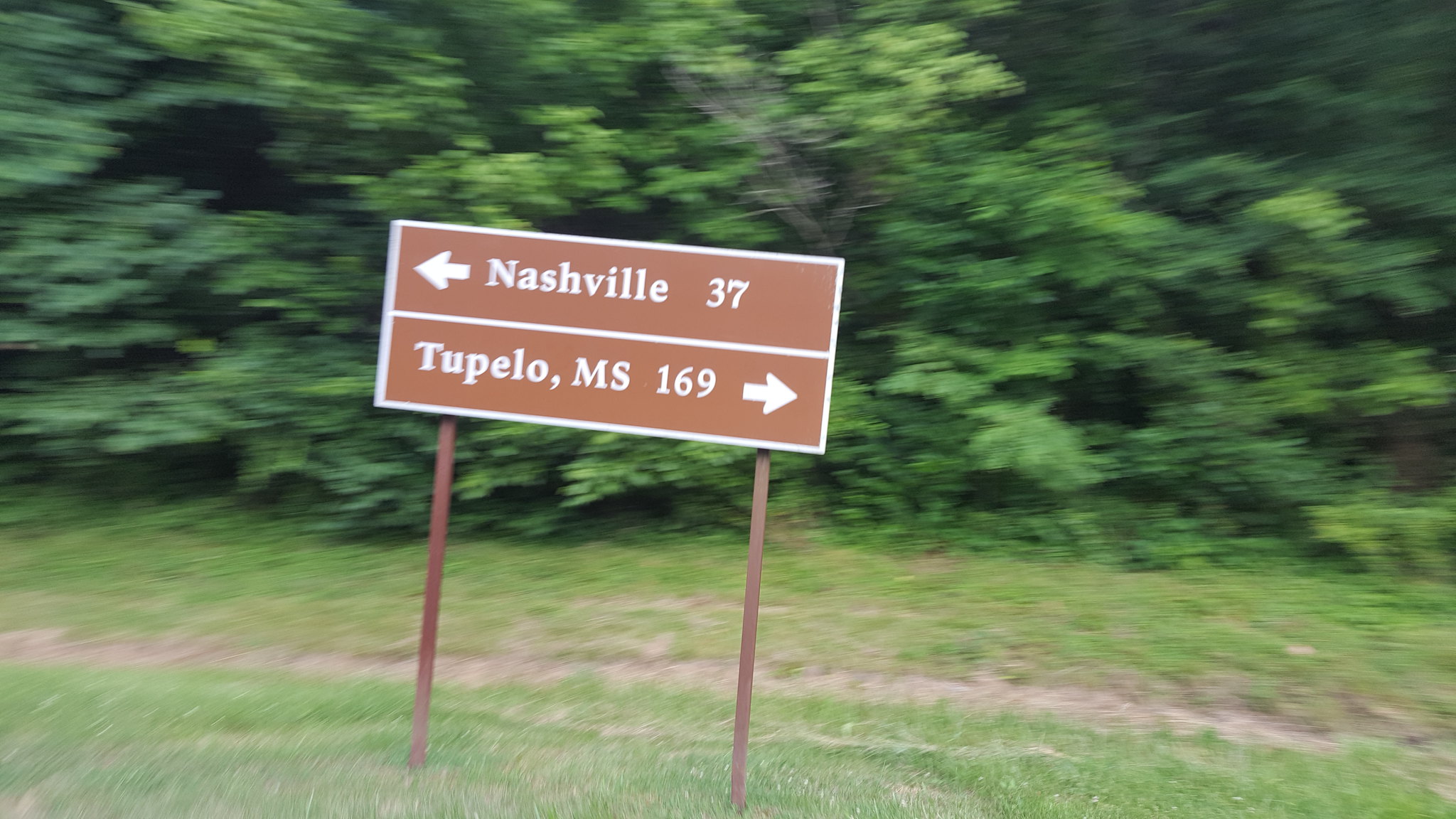A detailed color photograph, taken in landscape orientation, captures a directional sign at the side of a road. The photo was snapped from a moving vehicle, evident from the blurred trees and vegetation on the side of the road. The road itself is not visible, suggesting the shot was taken through a side window, as indicated by a slight reflection at the top of the image.

Despite the motion, the sign remains in sharp focus. It stands on two brown posts and is rectangular with a brown background. A white border frames the sign, which is divided by a horizontal white line. The top portion of the sign displays "Nashville, 37" with a white arrow pointing left, indicating that it is 37 miles to Nashville, Tennessee. The bottom portion reads "Tupelo, MS, 169" with a white arrow pointing right, showing a distance of 169 miles to Tupelo, Mississippi.

The grassy roadside appears freshly mowed, featuring a strip of cut, brown grass typical of a passing mower, and a drainage ditch runs horizontally across the scene. The contrast between the clear sign and the blurred background vegetation adds a dynamic element to the composition.